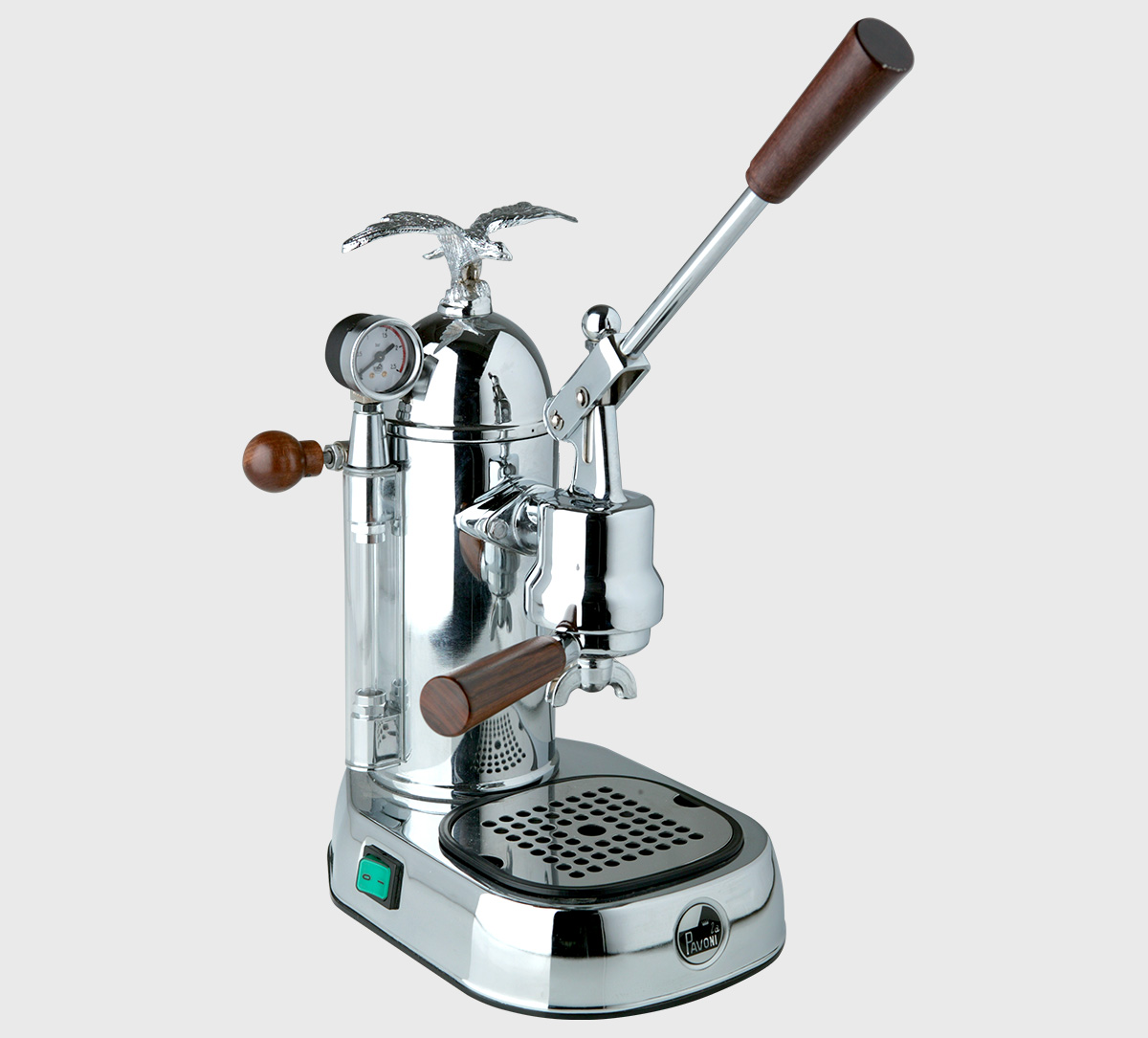The image depicts a detailed and elegant espresso machine with a predominantly silver, shiny aluminum finish. The background is stark white, accentuating the machine's sleek design. The machine features several brown wood-grain handles: three knobs, a tall lever in the front, and a handle where the espresso beans are placed. On the left side of the machine, there's a green power button, which appears to be in the on position. Toward the back left corner is a circular temperature gauge. The front of the machine has an L-shaped device positioned above a small black drip tray for placing cups, equipped with a cylindrical vertical piece at the back for stability. Additionally, the front bears the brand name "Pavoni," a tall, decorative eagle-like structure atop the machine, and a grated area at the base for liquid drainage. The entire appliance stands approximately a foot high, making a striking and functional addition to any kitchen counter.